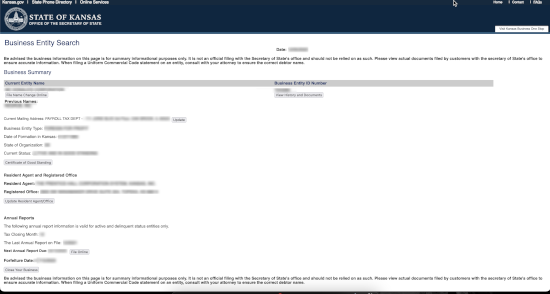This is a detailed screenshot of a website with a dark blue header prominently positioned at the top. Within the header, there are three distinct areas of white text located on the top left. The first reads "Kansas.gov," followed by a white separator. The second piece of text is too blurry to decipher, followed by another vertical separator. The third area of text reads "online services." 

On the top right side of the header, there are three lines of text, also separated by vertical white separators, but these lines are indistinct and blurry, rendering them illegible. 

In the bottom left section of the header, there's a white seal depicting a building encircled by a white ring. To the right of this seal, in bold white capital letters, is the text "STATE OF KANSAS," and beneath it, in smaller white capital letters, are the words "OFFICE OF THE SECRETARY OF STATE." Occupying the bottom right portion of the header is a white search bar containing light gray text, which is too blurry to read.

Separating the header from the page's body is a medium blue line. The main body of the page features a clean white background. 

In the top left corner of this section, blue text states "BUSINESS ENTITY SEARCH." Directly below this header, there are two lines of black text, but their content is too blurry to decipher. Just right of the center of the page, adjacent to the title, is a black word that is too blurry to be read, with a blurred gray bar of information to its right. The lower portion of the page contains multiple lines of text, many of which are obstructed by gray bars, making them indistinct and unreadable.